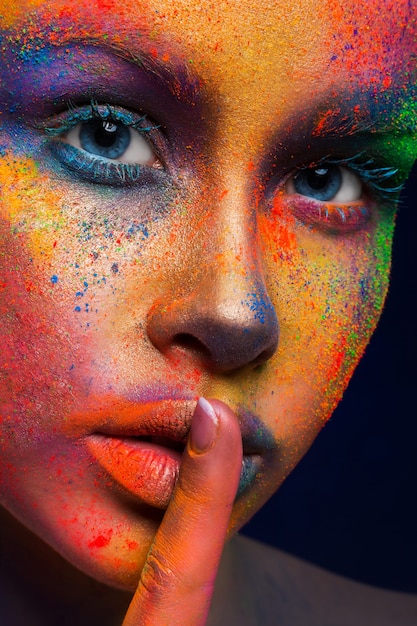This is a vibrant and intricate digital portrait of a Caucasian woman, featuring a close-up of her face adorned with an array of neon colors applied in a splotchy, spray-painted style. Her striking light blue eyes are complemented by blue-painted eyelashes. She holds her index finger over her lips in a quieting "shh" gesture. Her face is a canvas of vivid and varied hues - her forehead is painted gold, while the right side of her face is touched by orange and purple tones. Around her right eye, there is a burst of green, contrasting with the blue and purple swirls near her left eye. The left side of her face is dominated by orange-red shades. Her lips are equally colorful, with the left side painted orange and the right side purple. Set against a blue background, the image showcases her face, finger, and parts of her neck and shoulders, emphasizing the rich, vibrant colors that create an artistic and dynamic composition.